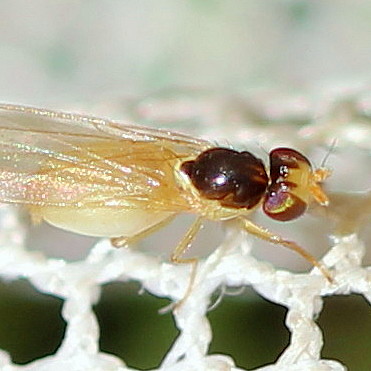The photograph showcases a close-up of a peculiar insect standing on a piece of white netting that features a hexagonal mesh design, resembling cotton. The insect's body is divided into distinct sections. Its head and forefront are dark brown, almost wine-colored, with light yellow accents and short, barely visible antennas. Its large, beady eyes are noticeable on either side of its head. The back section of its body transitions into a cream or translucent cloudy white color. The insect is detailed with four front legs and two back legs, all standing firmly on the netting.

Its delicate wings are translucent and glittery, capturing iridescent highlights in shades of pink, blue, and green. The thorax, situated between the wings, shares a purple hue reminiscent of an old plum. The overall impression of the insect is a mix of awe and unease, accentuated by its shiny, almost ethereal appearance against the blurred background.